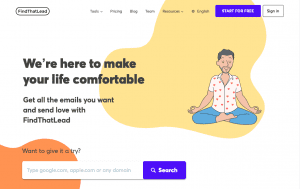This image is a horizontally-aligned screenshot of a web page featuring a large, clean white background. There are two abstract, circular blobs serving as design elements: a light orange blob situated in the lower left-hand corner and a yellow blob positioned towards the center-right. An illustrated man is central to the image, depicted in a meditative pose—sitting cross-legged with his fingertips touching. He is dressed in blue jeans and a white shirt adorned with red polka dots.

In the upper left-hand corner, the brand name appears, though it is illegible due to the low resolution. This section also includes some buttons or scroll bars, although specific details are unclear due to the image quality. The web page lacks a distinguishable banner, so headings are placed at the top of the page. These headings include "Tools," "Pricing," and "Shop," while others remain unreadable.

In the top right-hand corner, there is a purple sign-in button. The main text, located on the left side of the image, reads: "We're here to make your life comfortable. Get all the emails you want and send love with Find That Lead." Additionally, in the lower left-hand corner, superimposed over the orange blob, is the text: "Want to give it a try?" along with a search box featuring a purple search icon.